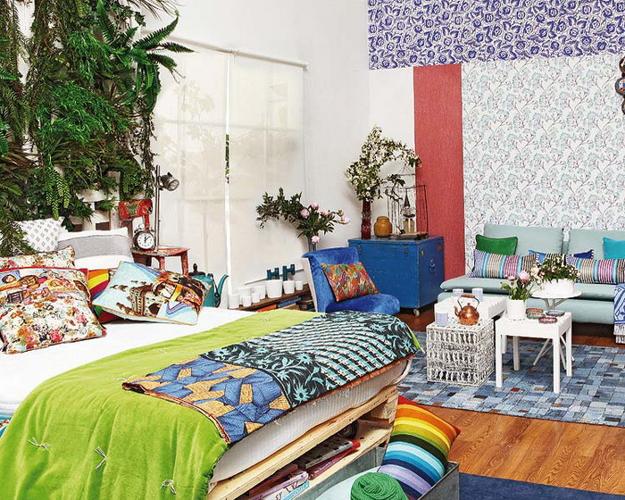The rectangular photograph captures an eclectic and vibrant bedroom with an array of colors and textures. Dominating the left side of the image is a large bed sitting on a brown wooden frame with a built-in shelf at the foot, filled with books. The mattress is covered by a white fitted sheet, layered at the foot with a green comforter and a blue and tan footrest blanket. The head of the bed is adorned with multiple squared pillows in various fabrics and prints, while the white wall behind it features hanging ferns and vines, giving a touch of greenery.

To the right of the bed is a window framed in white, allowing natural light to accentuate the room's lively decor. Below the window, there is a seating area featuring a couch decorated with several pillows. The hardwood floor is partially covered by a white and blue rug, on which sit two small white tables. One of these tables resembles white lattice and supports a flower vase, while the other table holds a bronze teapot.

In the bottom left corner of the image, near the bed, stands a blue cabinet displaying a vase with flowers and a piece of brown pottery. A blue velvet chair with a brown pillow is situated next to the cabinet, under an artificial tree. An attention-grabbing red nightstand near the bed hosts a clock and a light, further contributing to the room's quirky, non-matching aesthetic.

Overall, the room exudes an eccentric charm with its mix of colors, textures, and varied decor elements, underlined by a consistent white backdrop interrupted by hints of greenery and bursts of color.